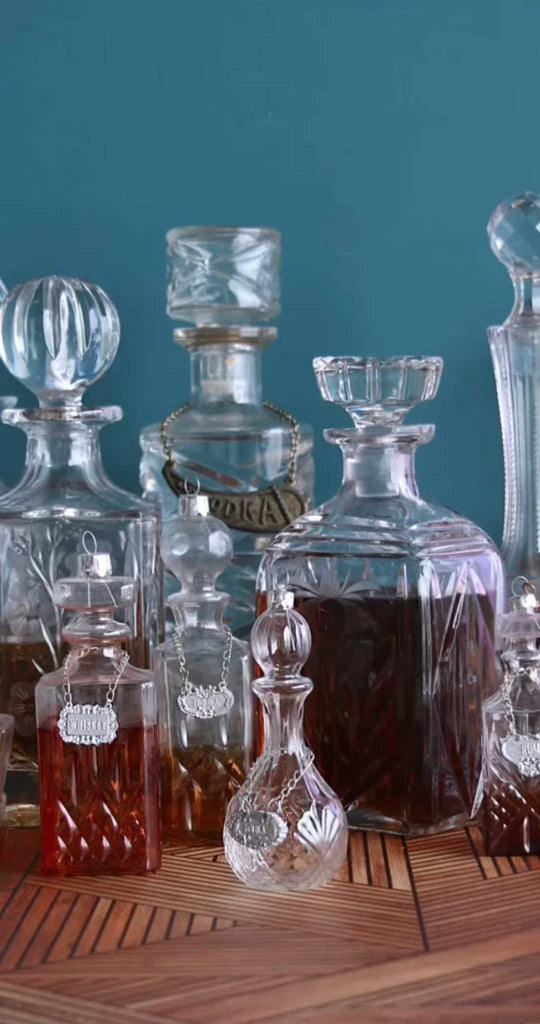The image depicts an exquisite collection of approximately seven or eight crystal decanters, each appearing to be meticulously hand-blown. These decanters, varying in shape and size, showcase a range of styles from tall and slender to wide and squat designs. Some of the decanters are half the size of others, adding to the visual diversity. Four of the decanters contain alcohol to varying degrees, with one prominently labeled as holding vodka. The decanters are adorned with silver and bronze chains and ornate tags, although most of the text on these tags is indecipherable.

In addition to their intricate carvings, some bottles feature unique lids equipped with hoops reminiscent of Christmas ornaments. The collection rests atop an intricately designed wooden table, its patterns complementing the elegance of the glassware. Behind the decanters is a dusty stone blue or dark teal wall, providing a rich, contrasting backdrop that enhances the opulence of the scene. This image captures not only the luxurious craftsmanship of the crystal decanters but also invokes a sense of refined aesthetic with its detailed and thoughtful composition.